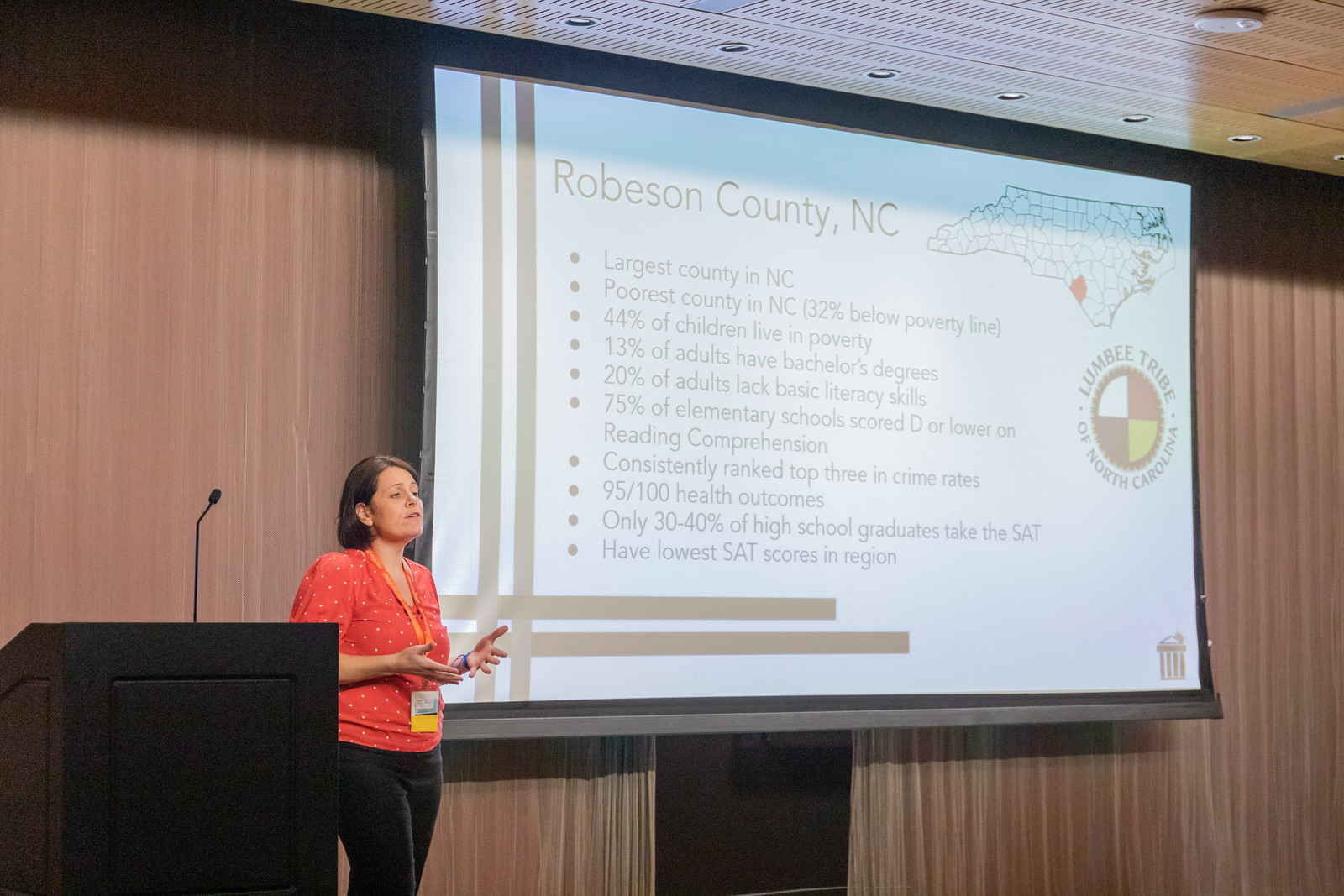This is a color photograph in landscape orientation capturing a woman giving a presentation on a stage beside a black podium with a microphone stand. The woman, who has shoulder-length dark hair, is dressed in an orange blouse with white spots and black pants; she wears a yellow laminated name tag around her neck. Her hands are outstretched in front of her as she addresses an audience not visible in the image. Behind her, a beige curtain frames a central projector screen displaying a slide with intersecting beige rules on its left and bottom. The slide is headlined "Robeson County, North Carolina" and features a highlighted map of North Carolina pinpointing Robeson County near the southeastern border. A circular logo with yellow and white opposing segments reads "Lumbee Tribe, North Carolina." The slide enumerates several statistical challenges faced by Robeson County: it is the largest and poorest county in North Carolina, with 32% of its population living below the poverty line; 44% of children live in poverty; only 13% of adults have bachelor's degrees; 20% of adults lack basic literacy skills; 75% of elementary schools scored D or lower in reading comprehension; the county consistently ranks in the top three for crime rates; it ranks 95th out of 100 in health outcomes; and only 30-40% of high school graduates take the SAT, with the county having the lowest SAT scores in the region. The photograph captures a moment of an educational lecture, possibly an initiative involving the Lumbee Tribe.